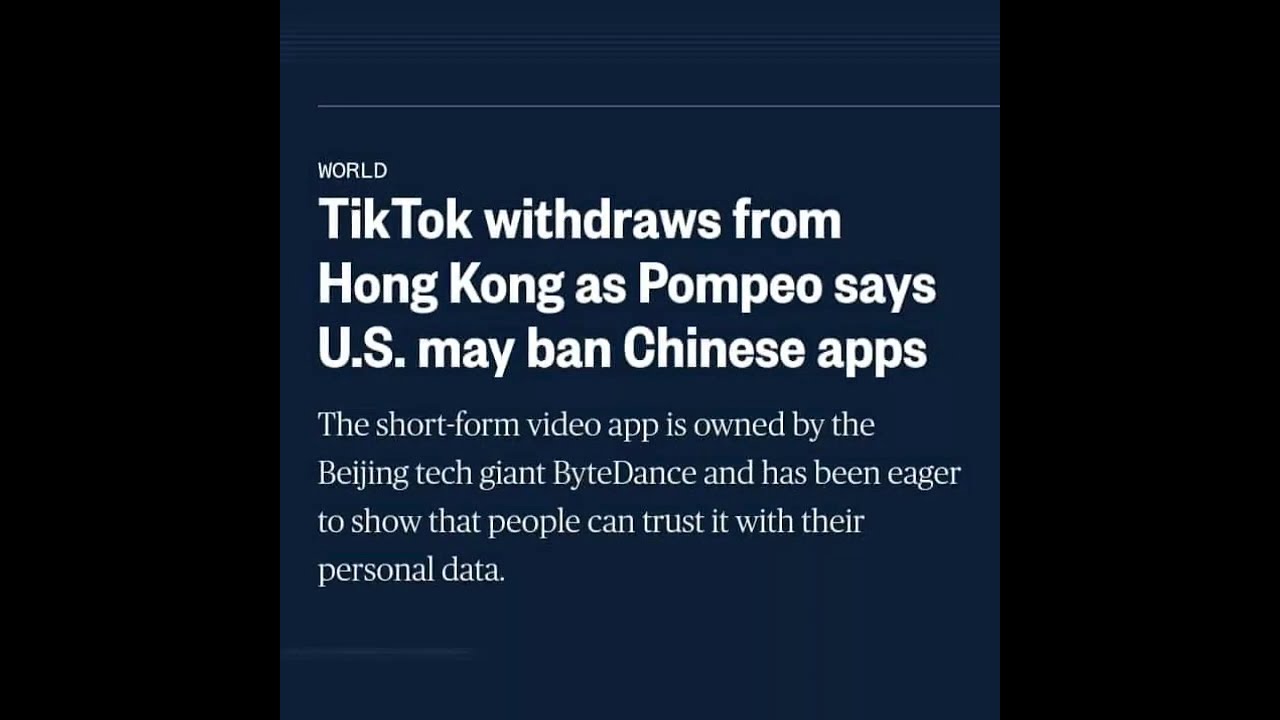This image is a cropped screenshot, likely taken from a mobile device based on its dimensions and the presence of black outer borders. The primary content is text with a dark navy blue background, originating from a news article. The article's headline reads "TikTok withdraws from Hong Kong as Pompeo says U.S. may ban Chinese apps," hinting at geopolitical tensions and regulatory actions. The subheading elaborates, stating, "The short-form video app is owned by the Beijing tech giant ByteDance and has been eager to show that people can trust it with their personal data." The article is categorized under "World News," as indicated in the top left corner. There are no images or additional visual elements in the screenshot; it is purely textual information.